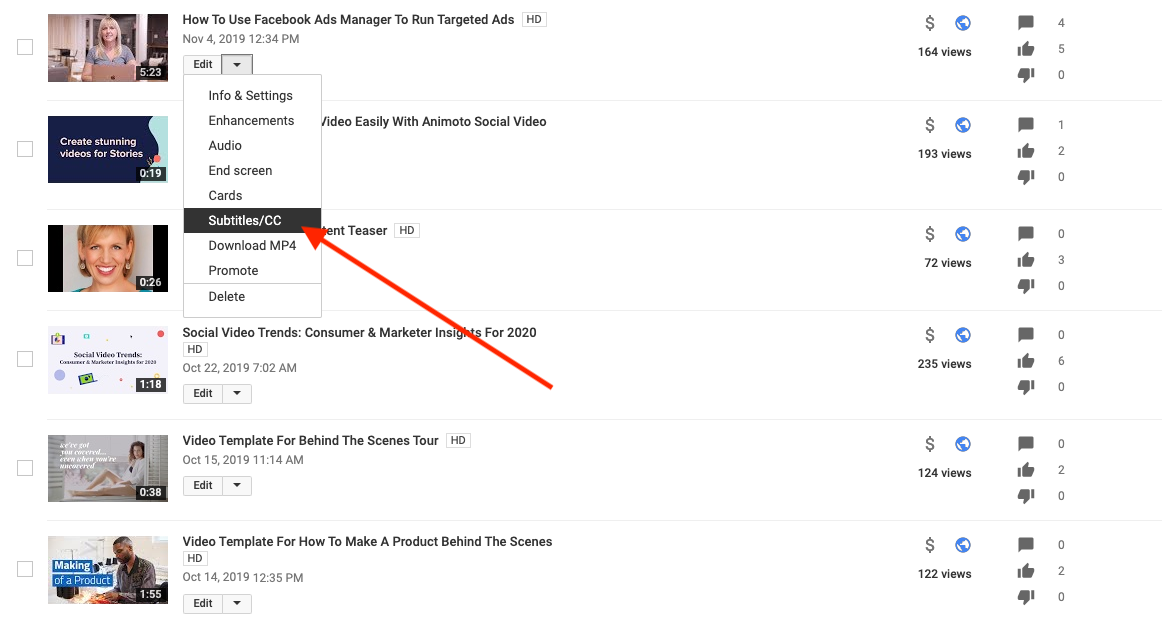This screenshot captures a webpage, likely from YouTube or Facebook, showcasing a list of video thumbnails arranged in six rows. Each row features a thumbnail image on the left, alongside details about the video's view count and its positive and negative ratings. A prominent diagonal red arrow points from the center of the page towards the upper left, directing attention to a tall, rectangular options box. This options menu includes various selections such as 'Info and Settings,' 'Enhancements,' 'Audio,' 'End Screen,' 'Cards,' 'Subtitles/CC,' 'Download MP4,' 'Promote,' and 'Delete.'

The videos listed cover a range of topics. Titles include: 
- "How to Use Facebook Ads Manager to Run Targeted Ads"
- "Social Video Trends"
- "Consumer and Marketer Insights for 2020"
- "Video Template for Behind-the-Scenes Tour"
- "Video Template for How to Make a Product Behind the Scenes"

The detailed structure suggests an emphasis on video content management and optimization tools, indicating a professional or enthusiast-level engagement with video production and marketing.